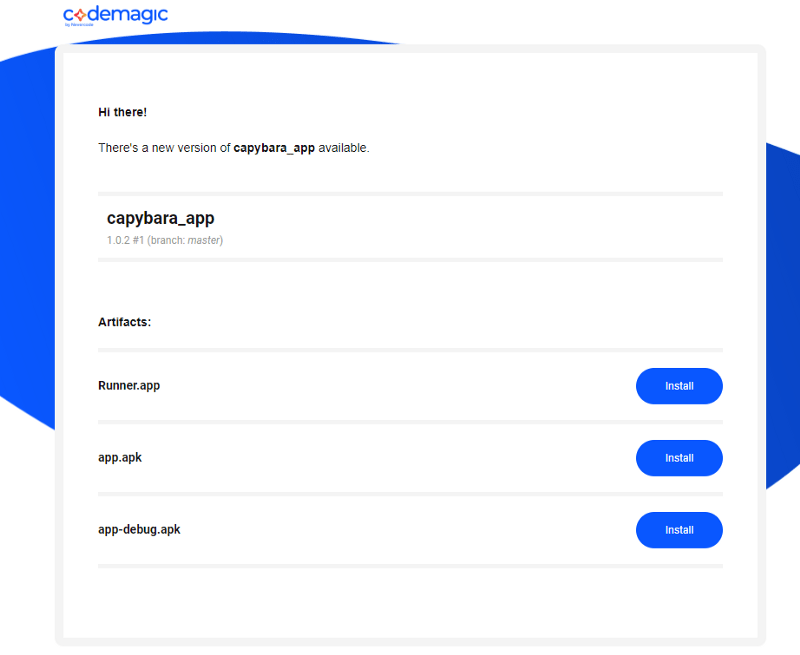The image depicts a user interface for a software development tool branded as Code Magic, indicated by the company's logo in the top left corner, which consists of a blue area featuring a small circular symbol for the letter 'O' accompanied by the text "Code Magic." Below the logo, a large central white box dominates the frame, displaying various elements and messages related to the application's functionality.

Overlapping the white box, a striking graphic element is incorporated into the background, featuring blue splashes that extend diagonally leftward across the top of the image. These splashes intermittently peek out from behind the large white box at the top left corner, the middle of the right side, and the left edge.

The white box's main content area includes a prominent message at the top declaring, "Hi there, there's a new version of Capybara app available. This is Capybara app." Beneath this message, the section labeled "Artifacts" is displayed, which enumerates three different application files: runner.app, app.apk, and app-debug.apk. Each of these files is associated with an "Install" button, allowing users to easily download and set up the respective applications.